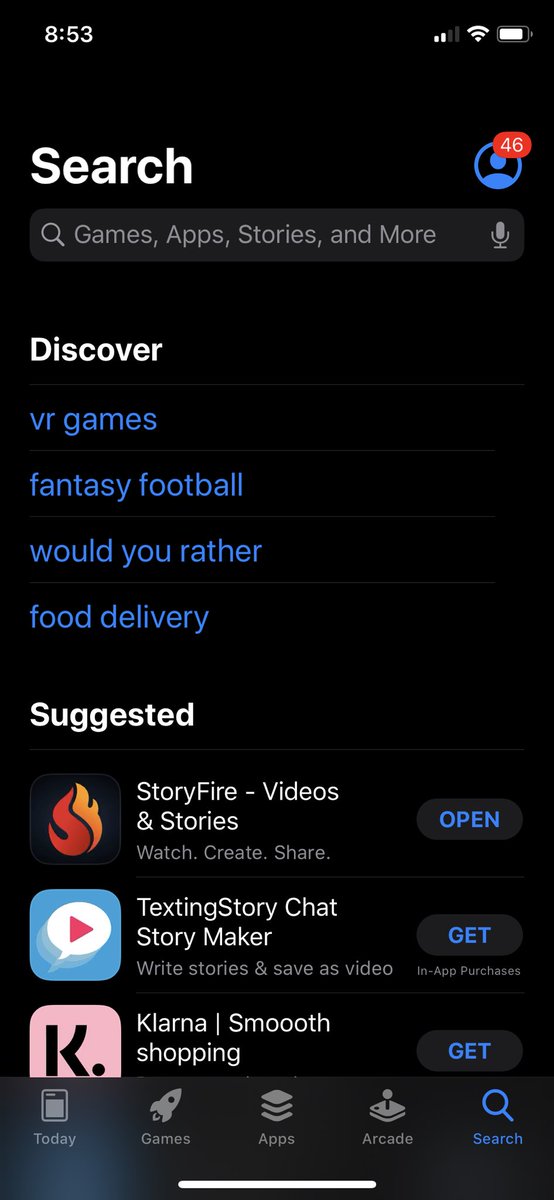This is a descriptive caption for the image you provided:

---

A screenshot taken from a mobile phone with a black background. The status bar at the top displays the time "8:53" on the upper left. In the upper right corner, there are two out of four bars of mobile signal, a full Wi-Fi icon, and a battery icon that appears to be fully charged. Below the status bar, in large bold white font, the word "Search" is prominently displayed. To the right of "Search", there is a small blue silhouette of a human within a blue circle, accompanied by a red square badge displaying the number "46" in white font.

Underneath, there is a gray search field with a magnifying glass icon, followed by the text "Games, apps, stories, and more". Adjacent to this field is a small microphone icon. Below this search bar, the word "Discover" is written in white font, followed by a horizontal white line.

Continuing down, various categories are listed, each separated by horizontal white lines. These categories include "VR Games" in blue font, "Fantasy Football", "Would You Rather," and "Food Delivery," each in white font. 

Further down, the section labeled "Suggested" appears in white font, with another horizontal white line beneath it. Below this line, there are some suggested applications, stories, and media titled "StoryFire - Videos & Stories."